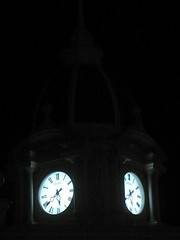This vertically-oriented, underexposed photograph captures an intriguing scene featuring two clocks set at a perfect 90-degree angle, appearing to be mounted within the same housing. The photograph's dark, possibly nighttime backdrop obscures many details, rendering the housing almost invisible against the pitch-black background. Despite the low lighting, the twin clock faces stand out, emitting a faint, possibly internal glow that accentuates their identical design. Both clocks feature clean white faces contrasted with classic black Roman numerals and hands, meticulously showing the time as 20 minutes to 6. The image evokes a sense of mystery and timelessness, leaving viewers to ponder the story behind these nearly hidden timepieces.